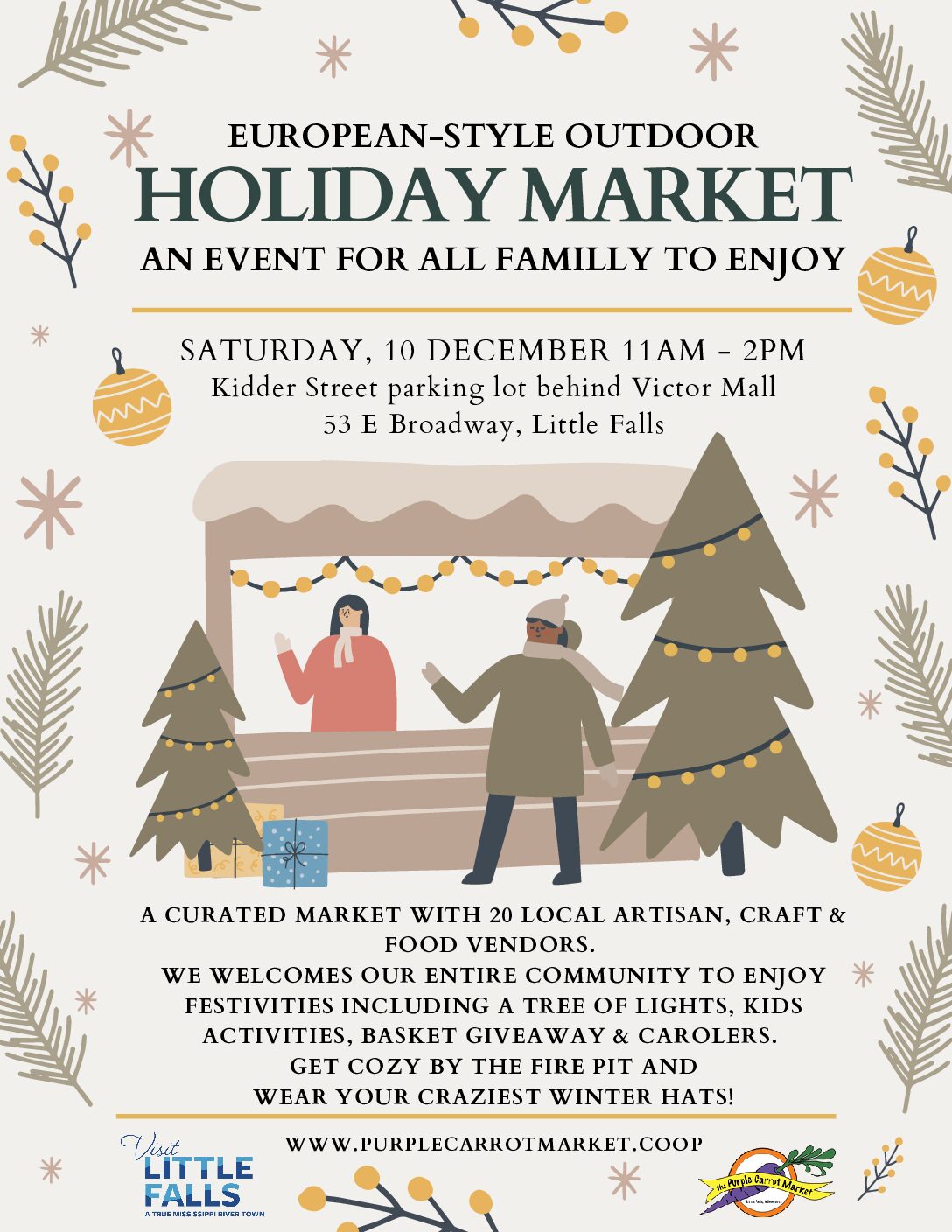This image is a vertically oriented white poster for a European-style outdoor holiday market. It advertises an event for the entire family to enjoy on Saturday, December 10, from 11 a.m. to 2 p.m. at the Keter Street parking lot behind Victor Mall, 53 E Broadway, Little Falls.

At the top, the key event details are prominently displayed, followed by a horizontal yellow line. Below this, there is an inviting illustration of a festive market stall. The stall features a vendor, possibly selling food items like hamburgers or hot dogs, interacting with customers amid a charming atmosphere. This scene is complemented by Christmas trees adorned with lights and decorations, alongside gift boxes scattered near the trees.

The poster is decorated with festive elements: clip art of Christmas trees, ornaments, starbursts, and spruce branches interspersed with snowflakes and Christmas bulbs. These decorations run along the borders and corners, giving the entire poster a cheerful holiday feel.

Towards the bottom, there is additional information about the vendors, activities, and a website link for more details. A logo for Little Falls is also included at the bottom, completing the festive and informative design of the poster.